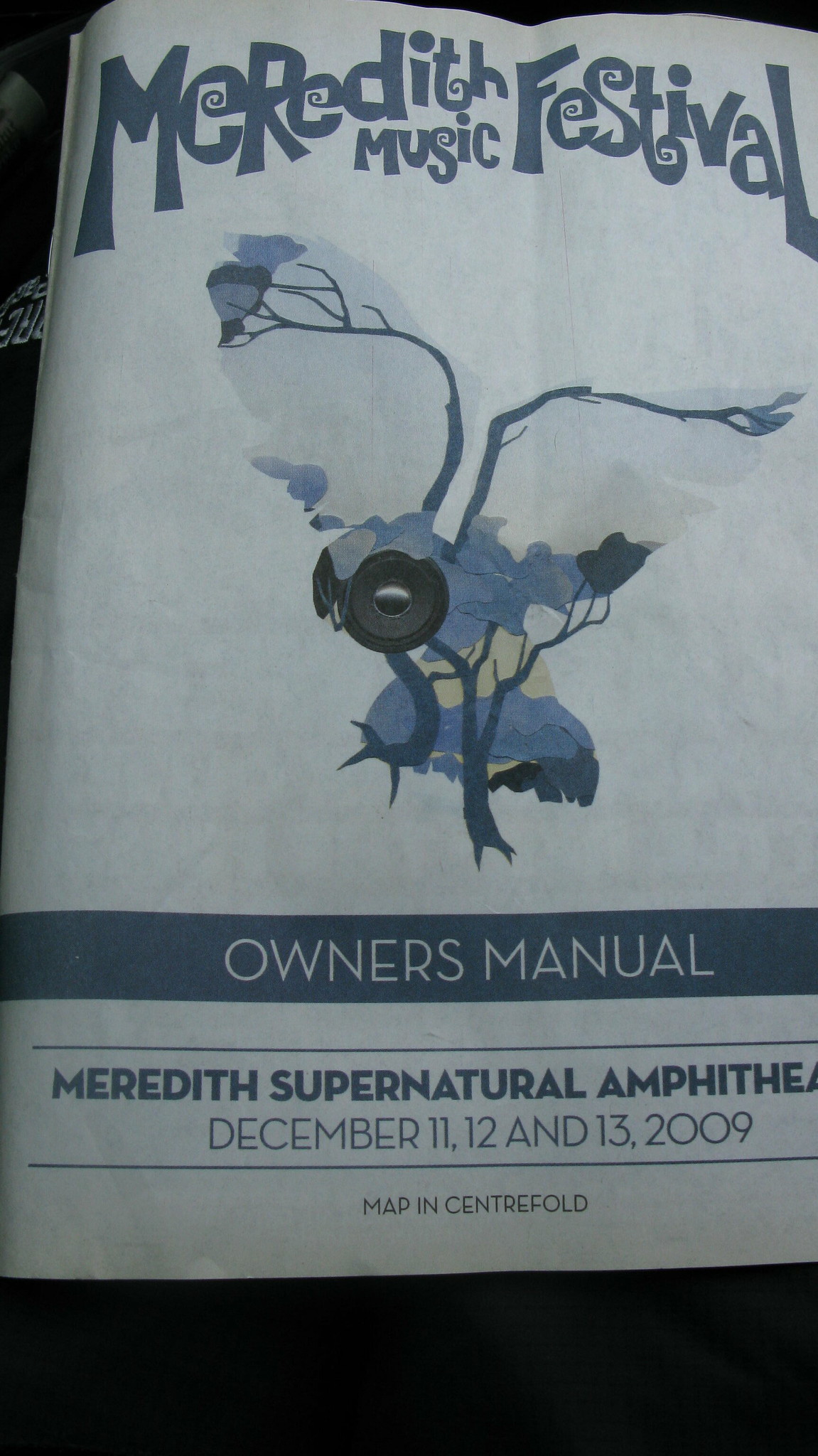The image is a flyer for the Meredith Music Festival, prominently featuring "Meredith Music Festival" in fancy blue font at the top. The letters 'E' in "Meredith" and in "Festival" have intricate swirls, as do the 'S' in "Music" and "Festival," contributing to the sophisticated design. In the middle, it reads "Owner's Manual," and at the bottom, it states "Meredith Supernatural Amphitheater, December 11, 12, and 13, 2009." A note indicates that a map is included in the centerfold for navigational assistance.

The flyer has a white background and includes a unique, digitally-drawn image of a bird. This bird is creatively designed to incorporate elements of nature: its wings resemble tree branches, and its legs morph into tree roots and trunk. The back of the bird shows hints of blue, emphasizing the blend of natural and drawn elements. The artistic style suggests a fusion of nature and digital art.